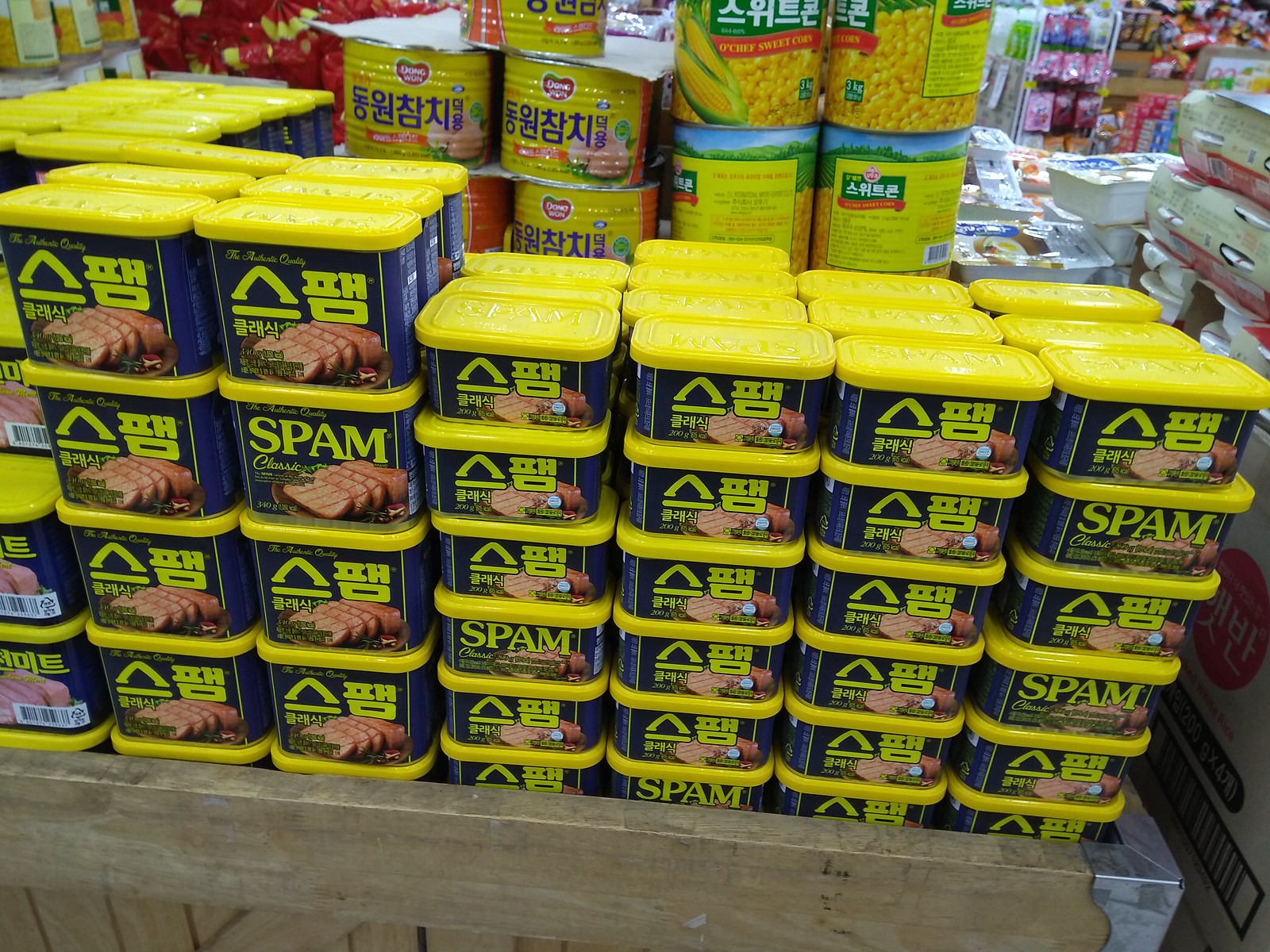In this landscape-oriented color photograph, we see a meticulous display at the end cap of an aisle within a bustling supermarket. The centerpiece is an impressive stack of rectangular cans of Spam, each dark blue can adorned with a bright yellow lid. The cans are arranged in a structured five-high and four-across formation atop a wooden crate reinforced with metal corners. The Spam cans prominently feature an image of grilled Spam slices along with the bold yellow word "Spam." Some of these cans have English labels, while others display the name in what appears to be Japanese, reflecting a bilingual packaging.

In the background, we notice another visually similar stack of canned food items, including what appears to be cans of corn, with labels entirely in an Asian script. Additional aisles of various grocery items stretch off to the right and left, with the supermarket's contents extending deep into the backdrop, emphasizing the scene's depth and realism. This vivid and detailed scene captures the essence of a typical supermarket's array, focusing on the internationally recognized Spam product displayed with a blend of cultural packaging.